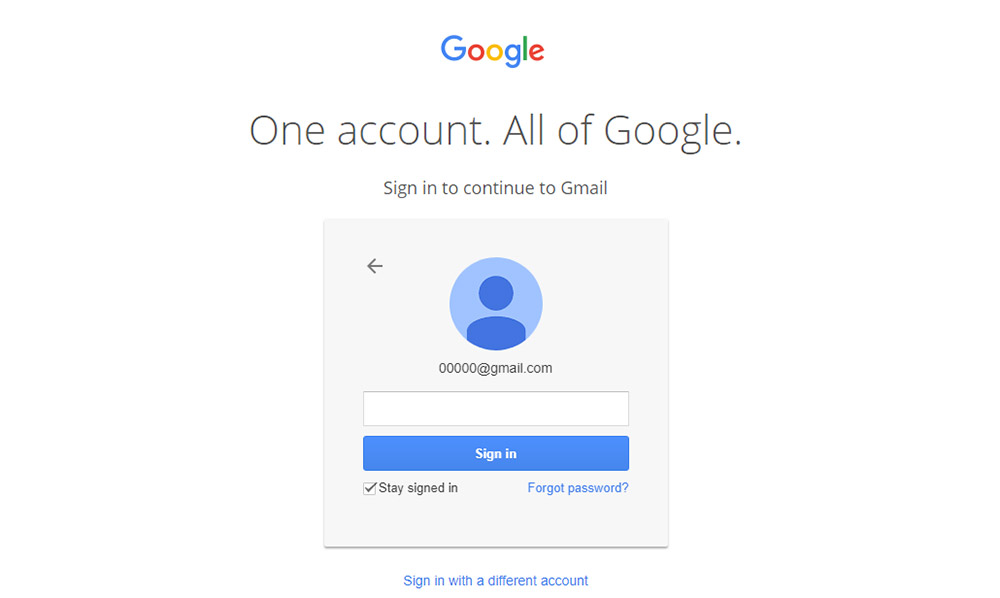The image showcases the Google Mail (Gmail) sign-in page, characterized by its clean and organized layout. At the top center of the page is the iconic Google logo, presented in its classic rainbow-colored font. Below the logo, a prominent message reads, "One account. All of Google," in large black letters. Directly beneath this heading, smaller text instructs users to "Sign in to continue to Gmail."

A light gray rectangular box is centrally displayed on the page, containing the login form. In the top-left corner of this box, an arrow points to the left, indicating a back or previous option. At the heart of the box is a circular icon with a light blue fill and a dark blue outline, suggesting a user's profile image placeholder. Directly below this circle, the placeholder text "00000@gmail.com" is shown, representing the email address field.

Beneath the email address field, there is a blank, horizontal white rectangle where users are expected to input their email addresses. Below this field is a blue rectangular button that prominently displays "Sign In" in white text, inviting users to proceed with their login credentials.

Towards the bottom of the login box, a small square checkbox labeled "Stay signed in" with a gray tick mark inside provides the option to remain logged in on the device. To the right of this checkbox, the text "Forgot password?" in blue serves as a clickable hyperlink for users who may have forgotten their login details. Further down, another blue text hyperlink reads "Sign in with a different account," offering an alternative login option.

The overall design is minimalistic, lacking additional extraneous text, ensuring that the user's attention is directed primarily towards the login procedure.